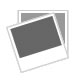A striking and detailed wall painting appears to be AI-generated and features the iconic figure of Darth Vader, emphasizing the interplay between light and darkness. The artwork is skillfully rendered in black and white, set against a light lilac-painted concrete block wall that provides a subtle yet contrasting backdrop. Focusing on Darth Vader's head, the painting captures the menacing essence of the character with precision. The familiar helmet, though not fully depicted, hints at its recognizable flared design around the cheeks. The dark, ominous eye sockets and the upside-down U-shaped nasal area are meticulously illustrated, leading down to the triangular mouthpiece adorned with a metallic grille-like pattern. Just beneath this, a slight hint of a collar can be discerned, adding to the realism and depth of the image. The combination of stark monochrome shades on a pastel background gives this AI-generated artwork a surreal and captivating presence.